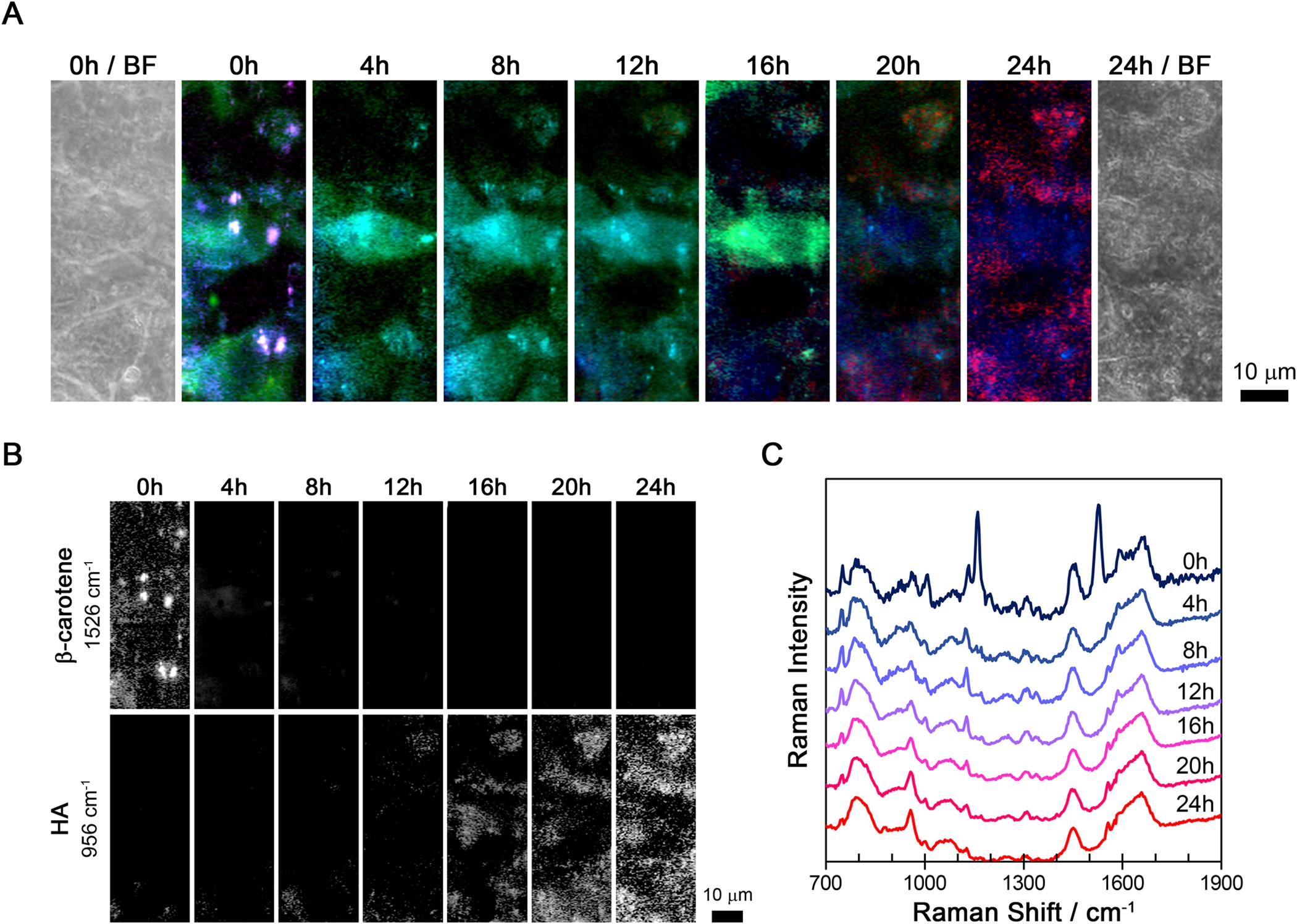The image is divided into three main sections labeled A, B, and C, each showing scientific charts illustrating data over a 24-hour period. Section A, occupying the top half, features a series of rectangular images labeled with time points: 0H, 4H, 8H, 12H, 16H, 20H, 24H, and 24H/BF. These images visually depict changes, becoming progressively darker as time advances, indicating some form of intensifying measurement, possibly fluorescence or another time-lapse phenomenon. Below A, section B on the bottom left consists of two subsections. The upper subsection represents changes in keratin, transitioning from scattered spots at 0H to a more solid appearance at 24H. The lower subsection shows HA, starting solid at 0H and progressively becoming rougher and more fragmented by 24H. Section C, located in the bottom right, presents a graph labeled "Raman Intensity," with the Y-axis detailing Raman intensity and the X-axis showing Raman shift in centimeters inverse. This graph tracks how Raman intensity varies across a 24-hour period, offering detailed shifts in spectral data.